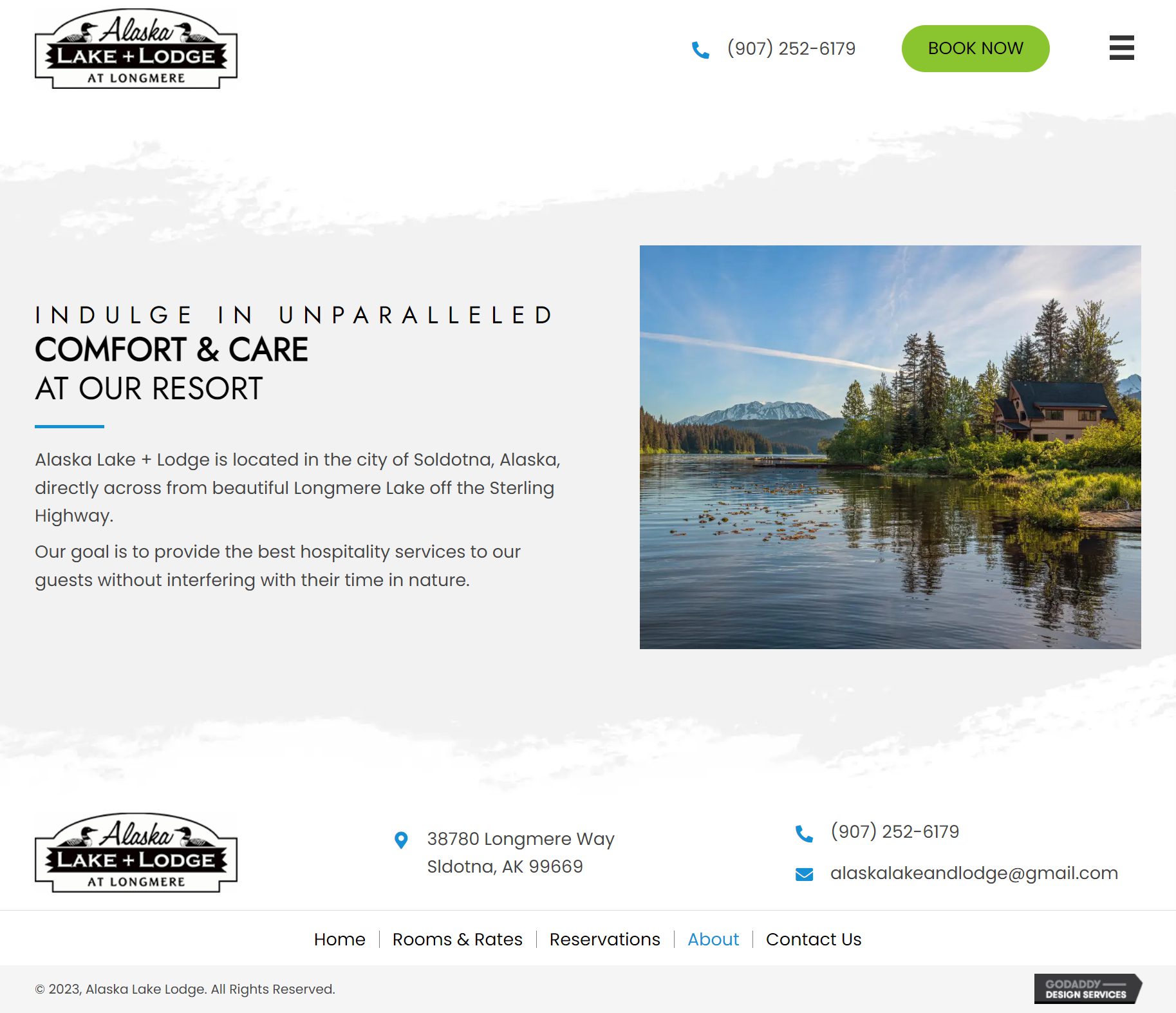Screenshot of a Lake and Lodge Hotel Website

The image captures a screenshot of the Alaska Lake and Lodge at Longmere's website. On the top left corner, the logo features two ducks flanking the word "Alaska," with "Lake and Lodge" displayed in white text against a black horizontal rectangle. On the top right side, a blue phone icon precedes their contact number (907-252-6197), followed by a green "Book Now" button. Adjacent to these is a three-line drop-down menu button.

Centrally, the webpage prominently displays the text: "Indulgent unparalleled comfort and care at our resort." Below, a description reads, "Alaska Lake and Lodge is located in the city of Sultona, Alaska, directly across from the beautiful Longmere Lake off the Sterling Highway. Our goal is to provide the best hospitality services to our guests without interfering with their time in nature." A picturesque photo of their lodge overlooking Longmere Lake complements this text.

In the bottom left corner, the logo reappears alongside a blue pin icon and their address: 38780 Longmere Way, Sultona, Alaska 99669. Below this, the contact number is repeated, and an email icon is followed by their email address: alaskalakeandlodge@gmail.com. The bottom section of the page includes navigation links for "Home," "Room and Rates," "Reservations," "About," and "Contact Us," with the "About" section highlighted in blue, indicating the current page.